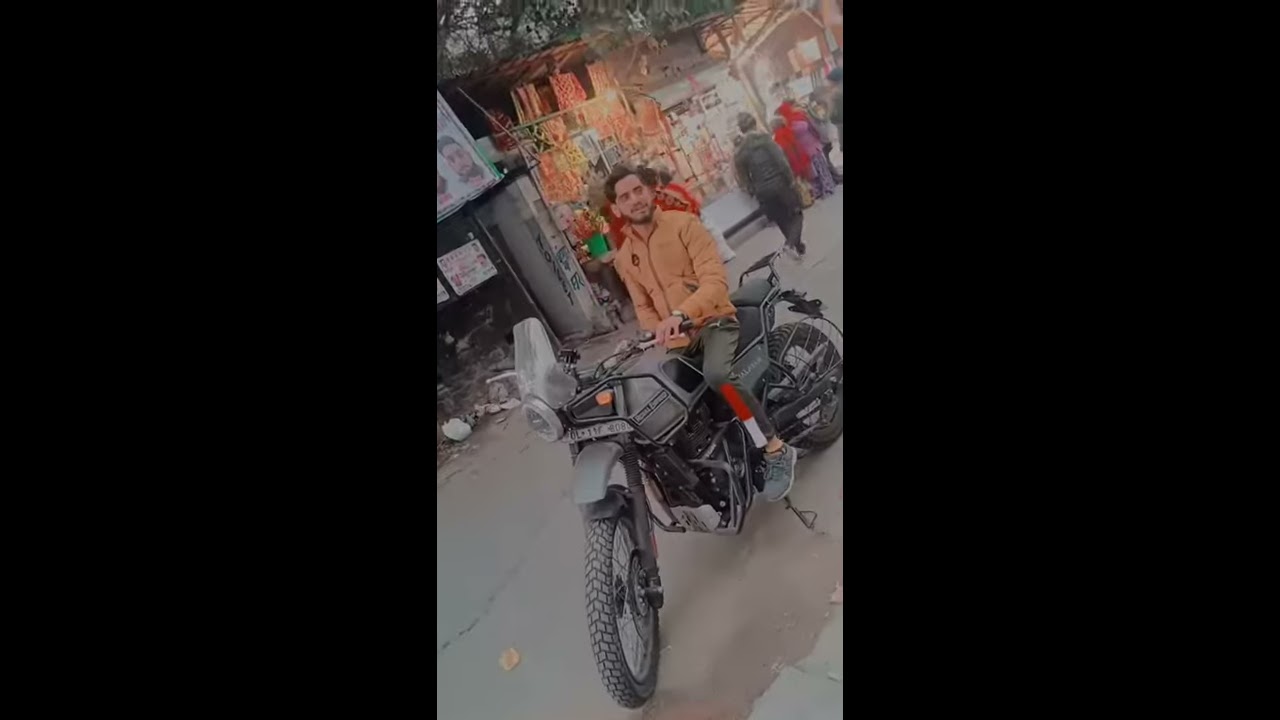This image captures a South Asian man with caramel-colored skin, short dark hair, and a black beard, sitting on a slightly beaten-up grey and black motorcycle, parked in the middle of a street. He wears an orange zip-up jacket and olive green pants with a distinctive red and white rectangle design on the leg. The motorcycle, possibly a dirt bike, has its kickstand down. The scene appears to be a less affluent area, suggested by the presence of temporary shacks or stands selling products, walls adorned with numerous posters, and noticeable trash and debris scattered around. Many people can be seen walking in the background, dressed in long-sleeve shirts and pants, indicating cooler weather. The photograph has a slight left tilt, with vertical black strips on both sides, adding to an impression that it might be a photo of a photo.